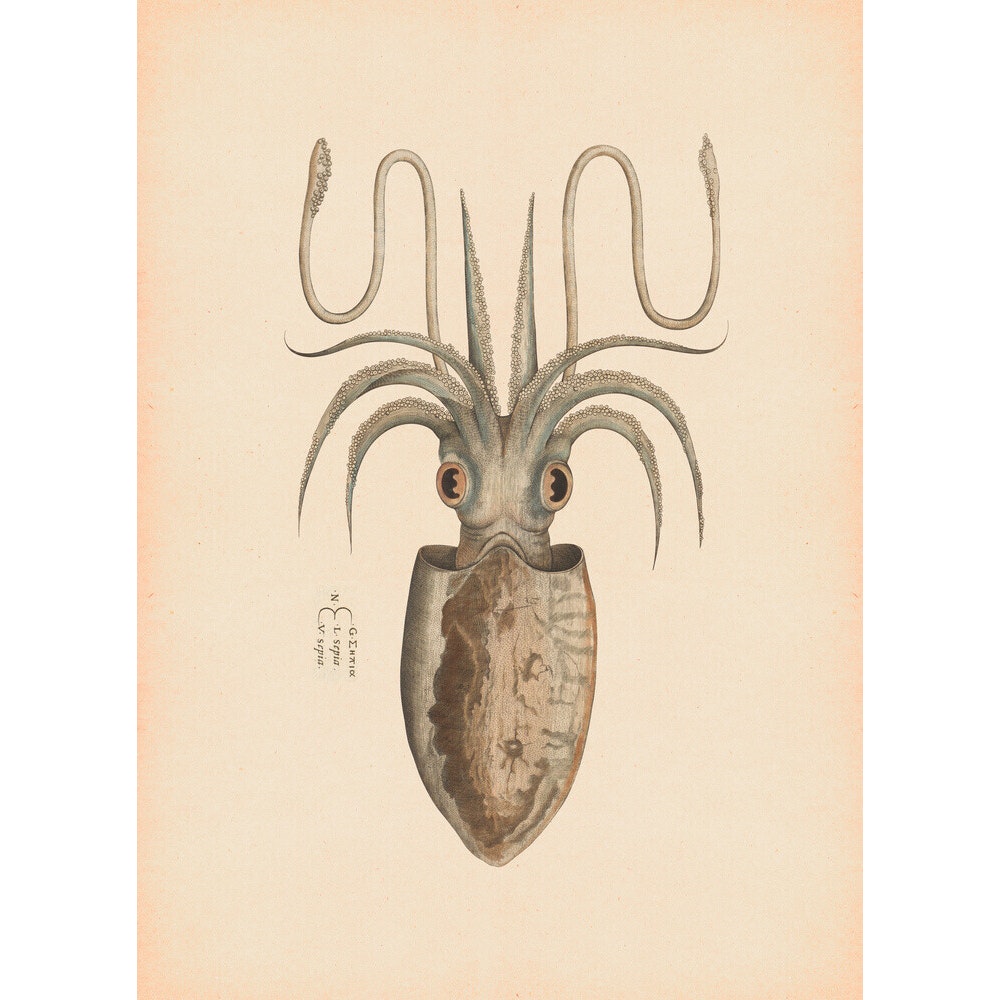The image is a rectangular illustration on a background edited to resemble vintage parchment paper, with its long sides being twice as lengthy as the short sides. The background features a gradient, starting with a tan color in the center that blends into a peachy tan as it reaches the edges. At the center of the image is a detailed drawing of a squid, oriented with its head downwards and its tentacles extending upwards. The squid, mostly depicted in light blue hues, has about ten tentacles: eight short and stocky ones, and two longer ones with bulbous ends. Its large yellow eyes are marked with black semicircles, giving it a striking appearance. Additionally, the lower part of the squid resembles an oval-shaped shell, adorned with a blend of white and brownish colors. Near the squid, particularly on the left side, is some small, illegible black text that includes Greek letters. This sophisticated and intricate sketch captures the essence of an unusual sea creature, blending real and possibly imaginary features in a striking manner.